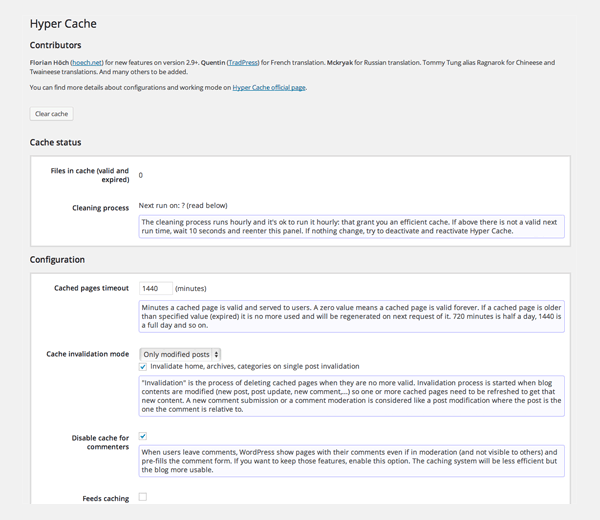Certainly! Here is a detailed and cleaned-up version of the descriptive caption:

---

At first glance, the image is a screenshot of a webpage filled with various details and settings related to cache management. The page features a light gray background with two prominent sections that stand out against their white backgrounds. The header identifies the content as pertaining to "HyperCache," a caching plugin for WordPress. Though blurry, the contributor names and their respective contributions are listed: 

- Florian Hilch (at hihoetch.net) for new features in version 2.9+
- Quentin Trade Press for the French translation
- Tami Tong (alias Ragnarok) for Chinese and Taiwanese translations
- Additional contributors to be added later

A blue hyperlink directs users to the official HyperCache page for more details about configurations and operational modes. Next to this link, a small box labeled "clear cache" is visible.

Below this, the "Cache status" section indicates that there are zero files in the cache, both valid and expired. The cleaning process is scheduled to run hourly, ensuring efficient cache operation. If the next run time is not valid, users are advised to wait 10 seconds and re-enter the panel, or deactivate and reactivate HyperCache if needed.

The "Configuration" section delves into specific cache settings. It starts with "Cached pages timeout," which is set to 1,440 minutes (one full day). This setting determines the validity period for cached pages, explaining that expired pages will be regenerated upon the next request.

The "Cache invalidation mode" setting, denoted by an up-down arrow, is set to "only modified posts." This section is enabled, indicated by a blue check mark, and it includes options to invalidate the home, archives, and categories on a single post invalidation. The term "invalidation" is explained as the process of deleting cached pages that are no longer valid, triggered by modifications to blog content such as new posts or comments. This ensures the cache is updated with the latest content.

Further, the option to "disable cache for commenters" is enabled, marked by a blue check mark. This setting ensures that when users leave comments, they see their comments immediately, even if those comments are still under moderation. This maintains user experience at the cost of slightly reduced cache efficiency.

Lastly, the "Feeds caching" option remains unchecked, indicating that feed caching is not currently enabled.

In summary, the image provides a comprehensive overview of the HyperCache plugin's configuration options for WordPress, allowing users to fine-tune their caching strategy to balance performance and user experience.

---